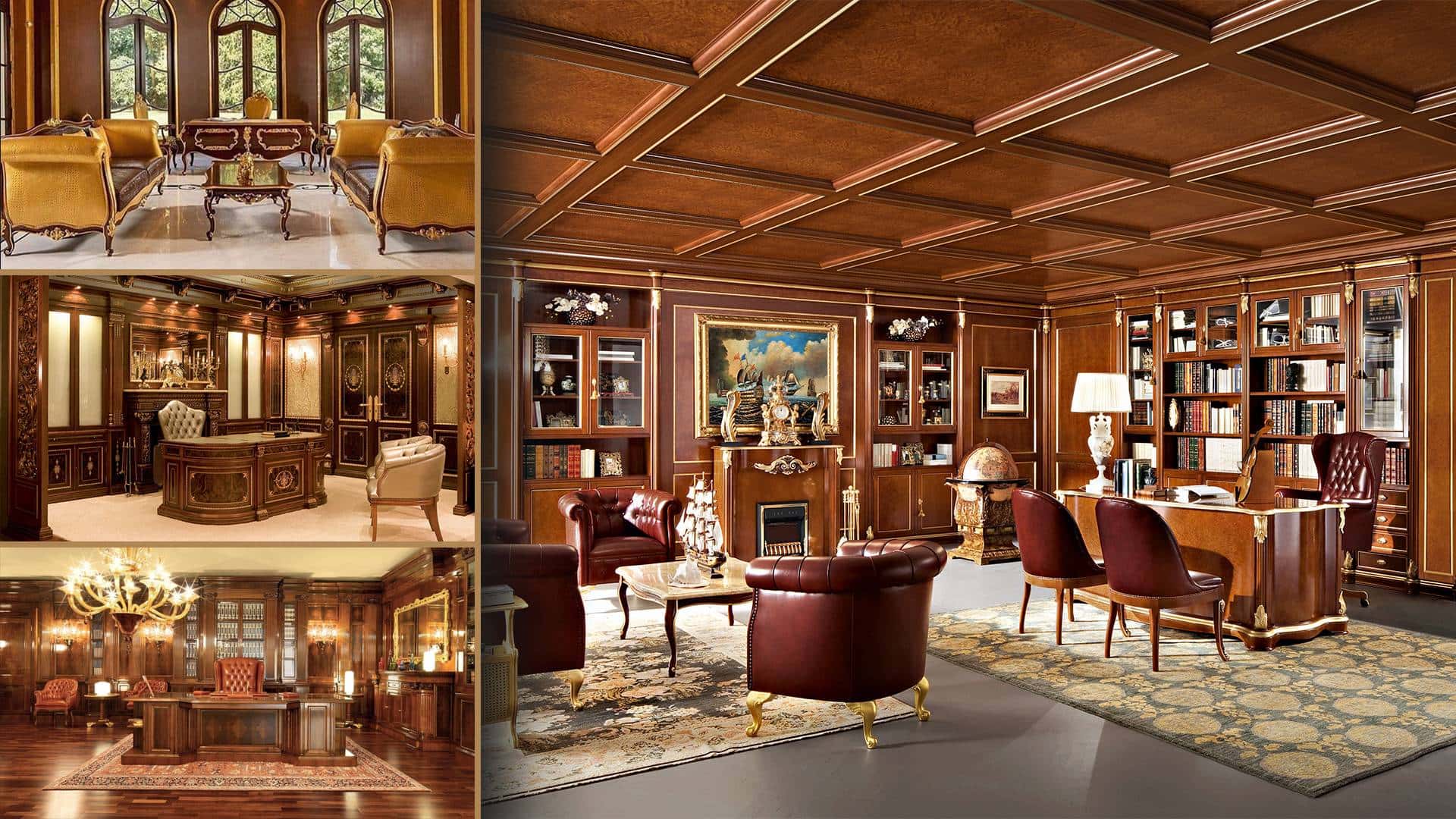The image showcases four meticulously designed executive office spaces, each embodying an opulent and uniform aesthetic with dark wood-paneled walls and ceilings. The main photograph on the right provides an expansive view of a wood-paneled room likely in a luxurious mansion or prestigious hotel, featuring built-in bookcases, multiple leather-backed chairs, and wood ceilings. There are three additional pictures on the left, each highlighting different areas within the same building, maintaining a cohesive design of rich browns, plush leather upholstery, and large, ornate windows. The top left image features gold-trimmed sofas with brown cushions, facing a coffee table, set against marbled floors and three large windows. Behind this setup, there's a desk with a chair. The middle left photo depicts a scene with wood paneling, a large desk, a red chair, and a plush carpet underneath. A chandelier hangs and hardwood floors extend throughout, adding to the room's grandeur. The bottom left image highlights another executive desk flanked by two chairs, set under a red carpet with an elaborate chandelier overhead, enhancing the luxurious atmosphere further. Each room employs strategically placed spotlights to showcase expensive furnishings, and the consistent presence of rich woodwork and leather indicates an overall theme of exclusivity and sophistication.